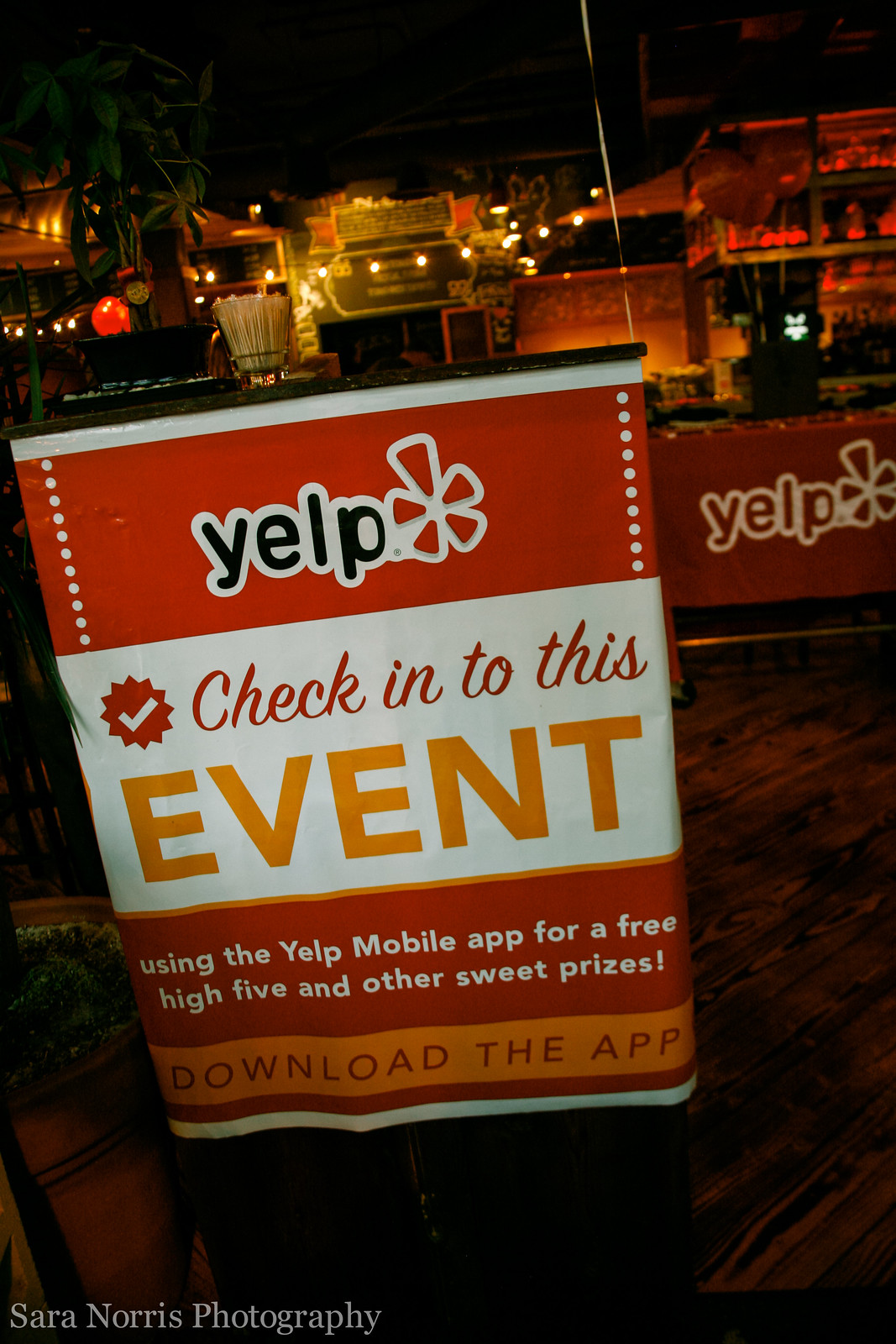The photographic image captures a bustling indoor convention hall, likely set up for a special Yelp event. Dominating the foreground is a vibrant banner, designed in red, white, and orange hues, featuring the prominent Yelp logo—a stylized red flower accompanied by a checkmark. The banner instructs attendees to "Check into this event using the Yelp mobile app for a free high-five and other sweet prizes. Download the app." Another identical banner stands adjacent, reinforcing the event's Yelp branding. The environment is dimly lit, with spotlights and warm orange tones illuminating a stage or possibly a movie screening area in the background. Below the bold banners, a watermark in the lower left corner credits "Sarah Norris Photography." Surrounding the space are elements that suggest a casual, festive atmosphere: a bar with an assortment of snacks, popcorn, and sodas, and a hostess stand equipped with a Yelp-branded podium and a jar of toothpicks. The eclectic mix of bar amenities and cozy restaurant tables indicate a versatile, multifunctional venue buzzing with activity and excitement.